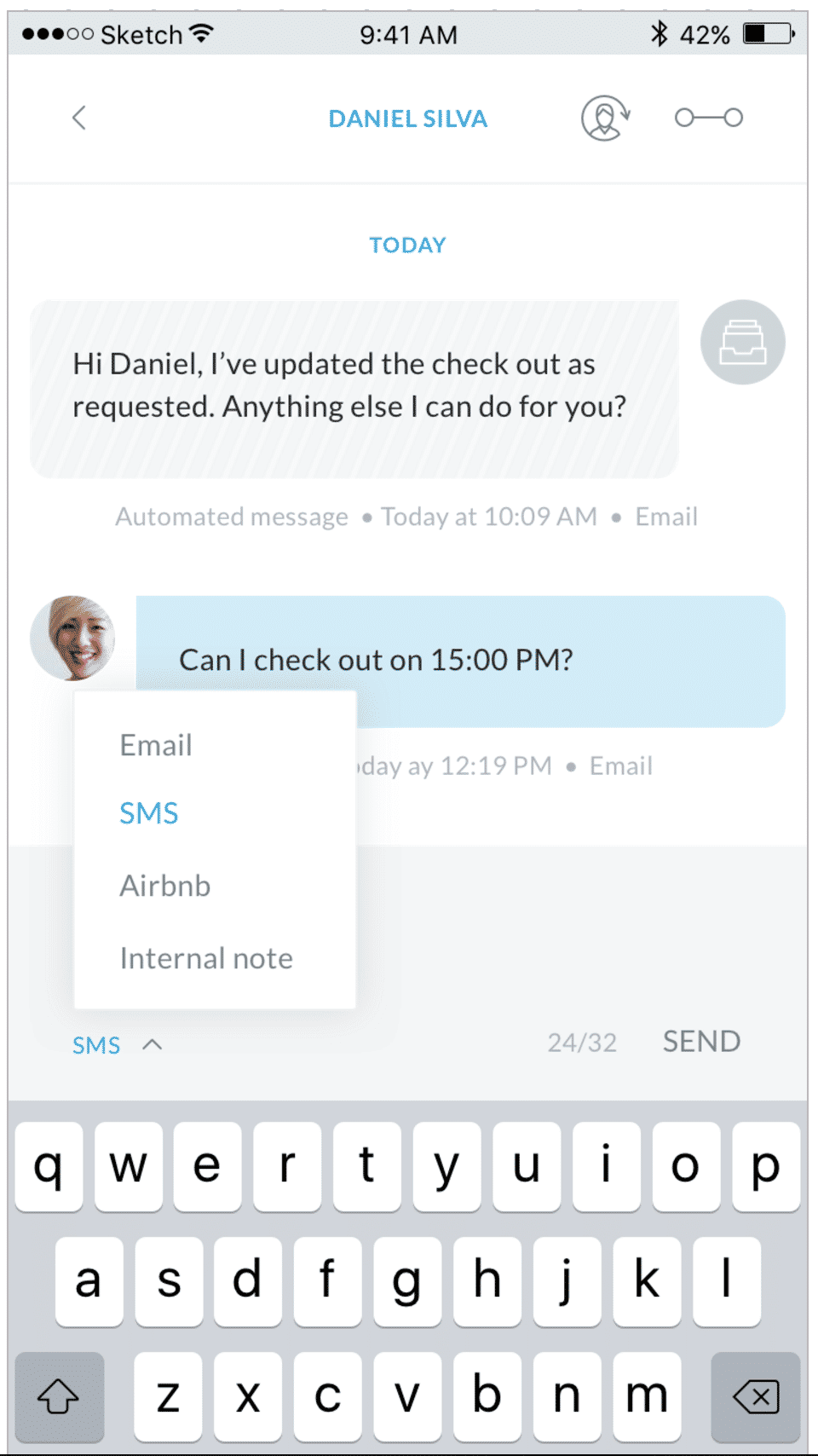A detailed caption for the image described could be:

"A screenshot captured on a mobile device at 9:41 AM displays a text message exchange. In the status bar at the top of the screen, the battery level is shown to be at 42%, and a signal strength indicator shows three out of five dots filled. The mobile's network provider is labeled as 'Sketch.' The background of the messaging app is white, and at the top, the sender's contact name 'DANIEL SILVA' is displayed in all capital letters and blue text. To the right of the contact name, there are icons representing a circular arrow and two circles connected by a line.

Beneath this header, the conversation displays a gray text box containing the message: 'Hi, Daniel, I've updated the checkout as requested. Anything else I can do for you?' This message is shown as sent by the other party. Below this, the reply from the phone owner appears in a blue text box: 'Can I check out at 15:00?' Adjacent to this reply, an avatar image of a smiling woman with short blonde hair and a gray background is visible.

Additionally, a small white menu is pulled up at the bottom of the screen, presenting four options: 'Email,' 'SMS' (highlighted in blue), 'Airbnb,' and 'Internal Note,' with the remaining options displayed in gray text."